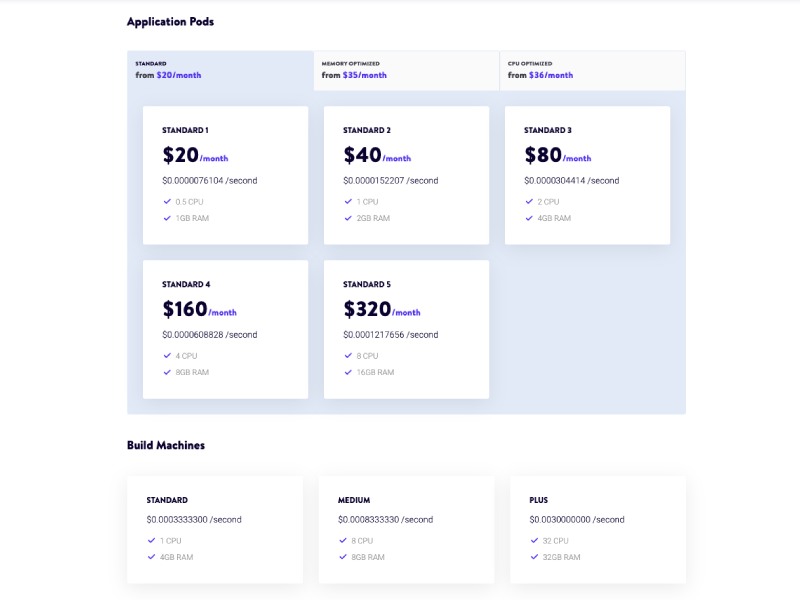The image appears to be a screenshot of a segment of a website, specifically showcasing various application pod plans and build machine options. 

**At the top**, there is a section labeled "Application Pods," separated by a gray horizontal line. This section includes three menu items:

1. **Standard**: $20 per month
2. **Memory Optimized**: $35 per month
3. **CPU Optimized**: $36 per month

**Below the menu items**, there are five informational cards arranged in a grid of three columns and two rows. The details on these cards are as follows:

- **First Row**:
  - **First Card**: 
    - Title: Standard 1
    - Price: $20 per month
    - Price Per Second
    - Resources: 0.5 CPU, 1 GB RAM
  - **Second Card**: 
    - Title: Standard 2
    - Price: $40 per month
    - Price Per Second
    - Resources: 1 CPU, 2 GB RAM
  - **Third Card**: 
    - Title: Standard 3
    - Price: $80 per month
    - Price Per Second
    - Resources: 2 CPU, 4 GB RAM

- **Second Row**:
  - **Fourth Card**: 
    - Title: Standard 4
    - Price: $160 per month
    - Price Per Second
    - Resources: 4 CPU, 8 GB RAM
  - **Fifth Card**: 
    - Title: Standard 5
    - Price: $320 per month
    - Price Per Second
    - Resources: 8 CPU, 16 GB RAM

The background of the cards is a light blue color.

**In another section at the upper left**, titled "Build Machines," there are three cards arranged in a single row with three columns:

- **First Card**:
  - Title: Standard
  - Price Per Second
  - Resources: 1 CPU, 4 GB RAM
- **Second Card**:
  - Title: Medium
  - Price Per Second
  - Resources: 8 CPU, 8 GB RAM
- **Third Card**:
  - Title: Plus
  - Price Per Second
  - Resources: 30 CPU, 32 GB RAM

This descriptive caption provides a detailed summary of both the application pod plans and the build machine options as showcased in the screenshot of the website segment.